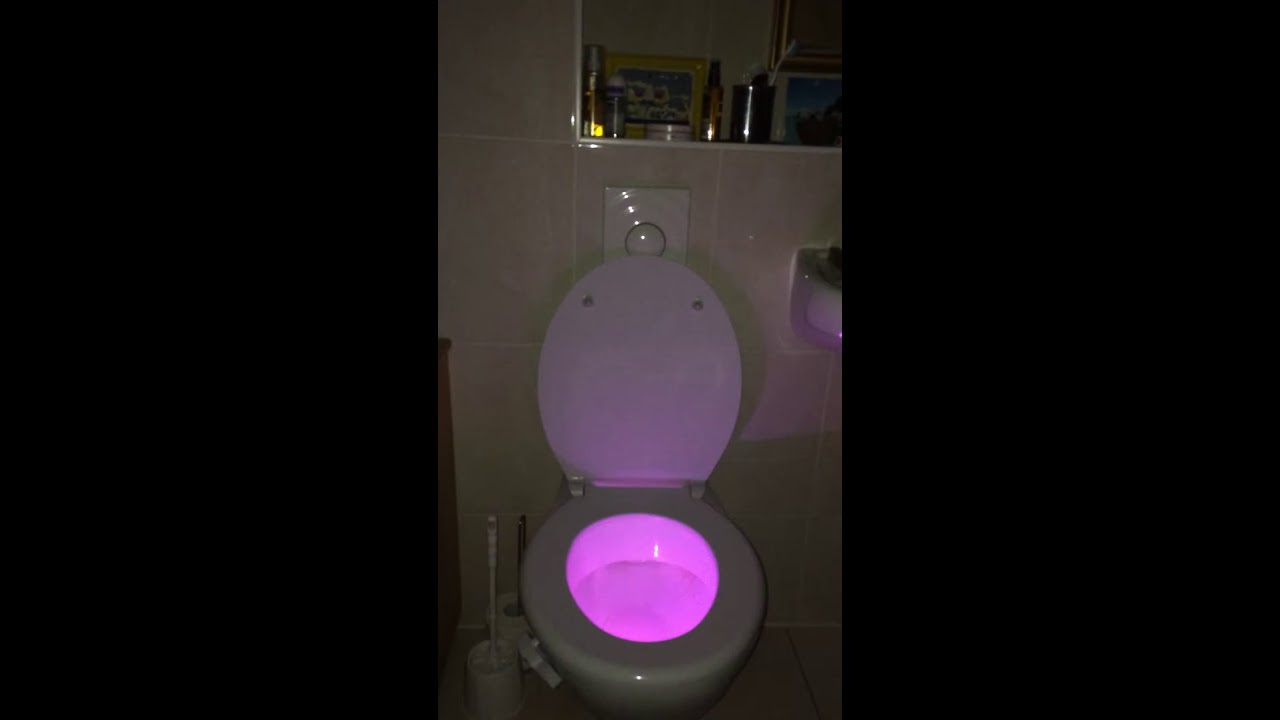The image showcases a bathroom with the lights off, highlighting a white, two-piece toilet positioned centrally. The most striking feature is the vibrant pink glow emanating from the toilet bowl, suggesting a neon light or other pink-colored illumination has been installed inside. This unusual pink underglow almost seems to pulse outward, drawing immediate attention.

In the background, the bathroom is decorated with light tan, shiny tiled walls and a white, glossy tiled floor. A shelf above the toilet holds various bottles, likely perfumes, hairspray, and cologne, along with a silver cup that appears to be a toothbrush holder. Three pictures lean against the back of this shelf, adding a personal touch to the otherwise utilitarian space. Additionally, a small white sink is visible to the left of the toilet, while toilet brushes and cleaning supplies are placed nearby, further contributing to the practical ambiance of the bathroom.

The flush mechanism is integrated into the upper part of the ceramic shelf behind the toilet, hinting at a European design. This carefully detailed image uniquely captures the intriguing blend of aesthetics and functionality, underscored by the captivating pink illumination in the toilet bowl, designed for nighttime convenience without the need to switch on the main bathroom lights.